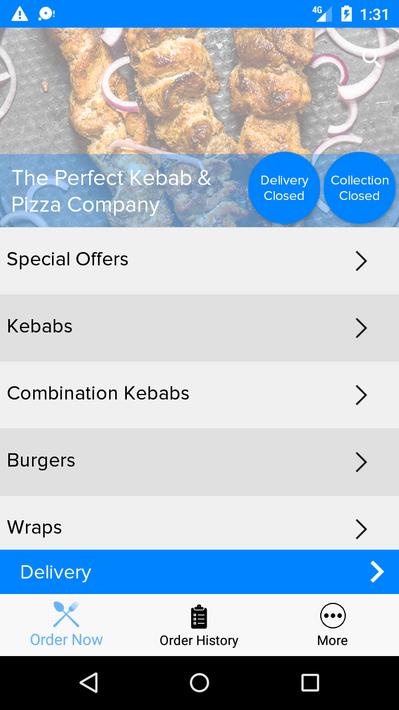The screenshot showcases a user interface of a food delivery application. 

At the top of the image, there is a bright blue banner featuring a blue triangle with a white exclamation mark, a round circle, and a battery icon with a lightning bolt, all positioned towards the left. Towards the right, it displays "4G" alongside a cell signal icon with a "Y" symbol, and the time, which is 1:31.

Below this, a graphical section features images of onions and other food items. Overlaying the image is a clear light blue banner with white text that reads "The Perfect Kebab and Pizza Company." Adjacent to this, two blue circles display messages in white text: "Delivery Closed" and "Collection Closed".

Following this, the screen alternates between lighter and darker beige sections. The light beige section lists "Special Offers" with arrows pointing to the right. This is followed by options for "Kebabs," "Combination Kebabs," "Burgers," and "Wraps" in similar alternating beige tones.

Further down, a blue banner in white text indicates a "Delivery" section with a right-pointing arrow, followed by options such as "Order Now," "Order History," and "More."

At the very bottom of the screen, there is a black navigation bar featuring three icons: a left-pointing arrow, a circle, and a square.